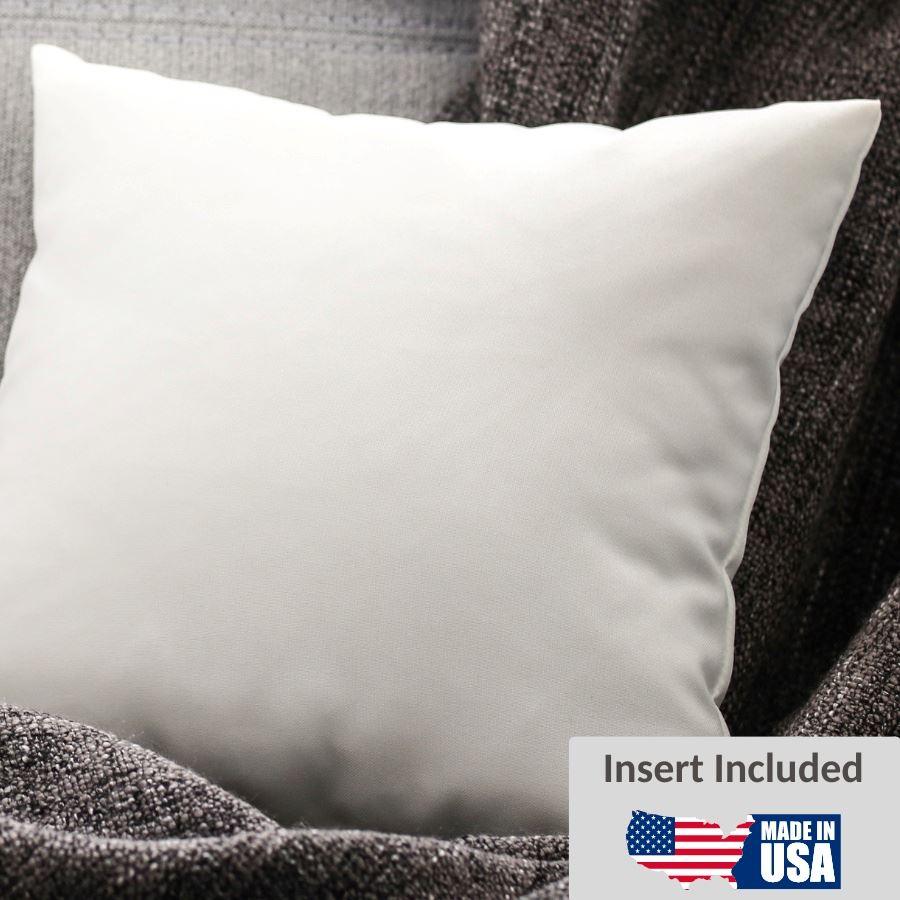This image features a single, square-shaped throw pillow prominently positioned in the foreground, suitable for a sofa or chair. The pillow has pointed corners and displays some distinct wrinkles along its right side and bottom edge, adding a touch of texture to its appearance. Behind the pillow, a draped piece of dark gray cloth, likely wool, creates a cozy yet sophisticated background. Additionally, a lighter gray cloth is subtly visible further behind, enhancing the layered textile setting. In the bottom right corner of the image, there is a gray rectangular label showcasing an American flag-inspired symbol, prominently featuring the map of the United States in red, white, and blue, complete with a blue corner adorned with white stars. The label reads, "Insert Included. Made in the USA."